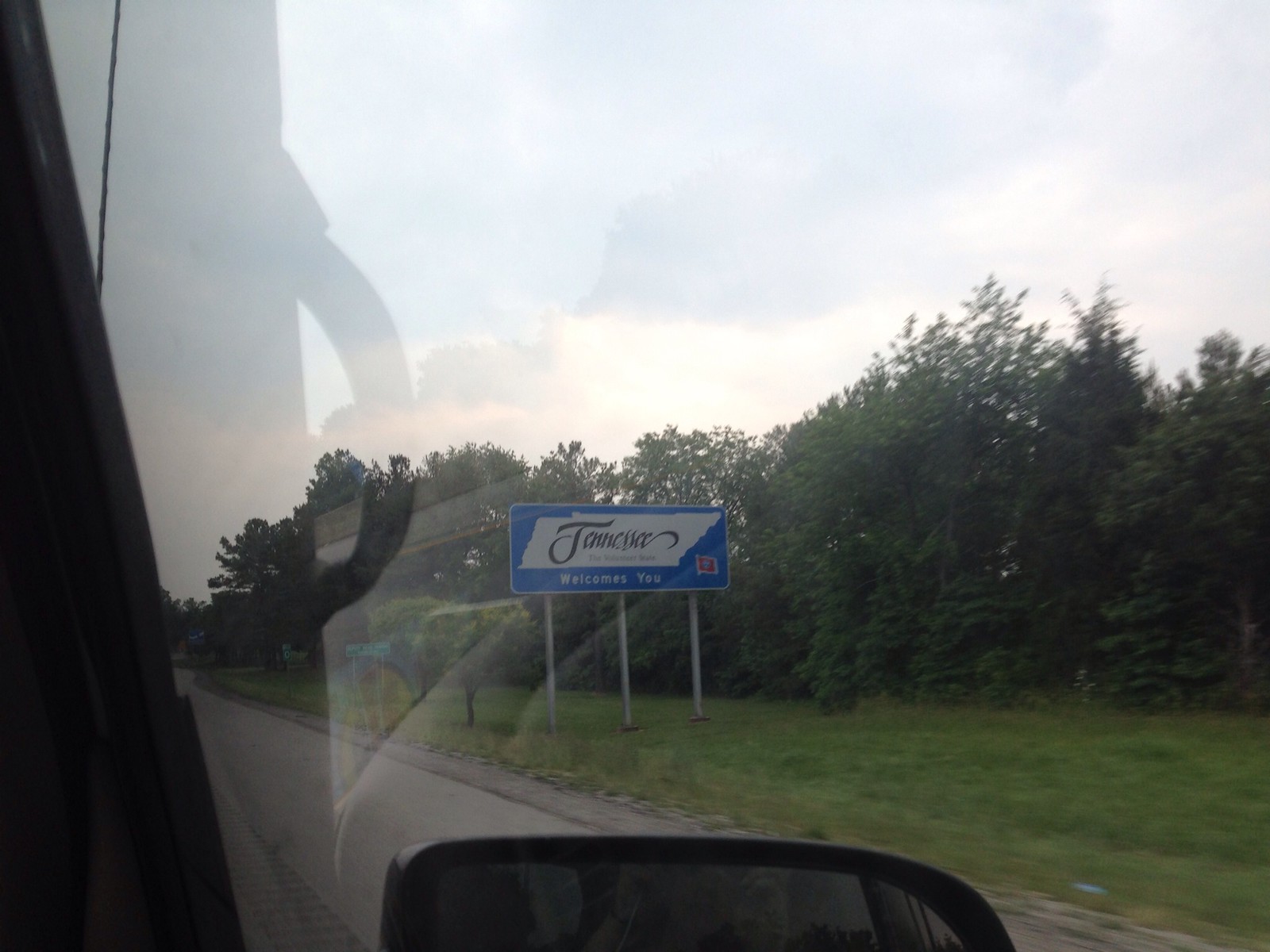A photograph taken from the passenger side of a moving vehicle captures a partial view of a black car door and rearview mirror, reflecting the car's interior handle. Outside the vehicle, the camera captures a scenic, lightly wooded roadside. Prominently featured in the composition is a blue sign adorned with a white silhouette of the state of Tennessee and black lettering that reads "Tennessee Welcomes You."